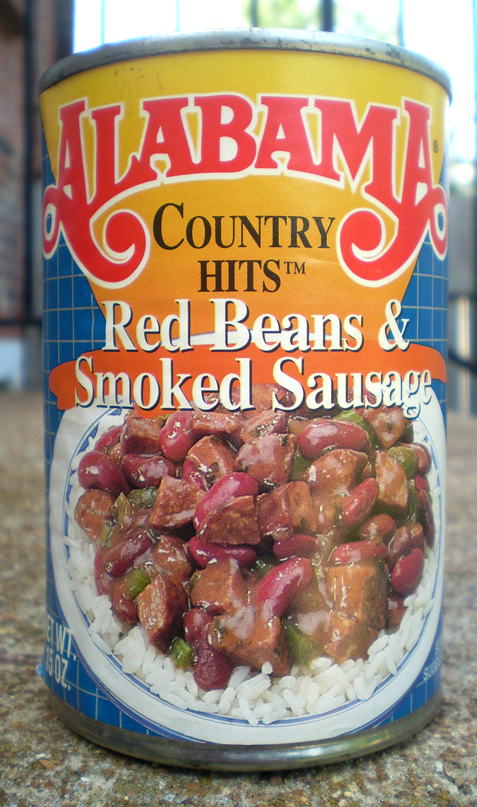The image showcases a can of "Alabama Country Hits Red Beans and Smoked Sausage" prominently displayed on a stone or marble surface that is a mix of brown, grey, orange, and white colors. The can itself features a striking design with a blue label overlayed with a bronze square grid pattern. The top and bottom rims are silver, and the label is bordered with a yellow trim. At the top of the label, an upside-down yellow triangle contains the word "Alabama" in red lettering with a white outline, and just below it, "Country Hits" in black with a small trademark symbol. Further down, "Red Beans and Smoked Sausage" is written in white letters. The label includes an appetizing image of the dish: a bed of white rice on a white plate with a blue design, topped with red beans, chopped brown sausage, a savory sauce, and bits of chopped green onion. The scene appears to be set outdoors, possibly on a porch or patio, with a black metal railing and a glimpse of a brownish-red brick building, a bright blue sky, and green tree leaves in the background.